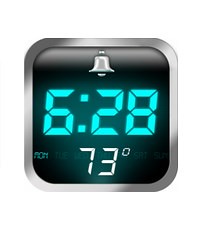This is a highly detailed, computer-generated image of an impeccably designed digital clock, showcasing its precise and polished appearance that could only be achieved with the aid of advanced computer software. The clock features a square shape with gently rounded corners and is encased in a medium-width, silver-colored border that adds a touch of modern elegance.

Dominating the design is the black screen, which occupies the central portion of the clock's face. The digital readout is prominently displayed, occupying the upper half of the screen with digits that are illuminated in a soft, light blue hue, currently showing the time as 6:28. 

Directly above the time display, centrally located, is a clear image of an alarm clock, indicating that the alarm function is activated. Below the current time, there is a day indicator, which can display days from Monday to Sunday. The abbreviation "MON" is specifically highlighted in a matching light blue color, signifying that today is Monday.

Further enhancing the informational layout, beneath the day indicator, a temperature reading of "73°F" is presented in crisp white text, providing a quick reference to the current ambient temperature. Overall, this digital clock blends functionality and aesthetic appeal seamlessly, making it both a practical tool and a visual delight.